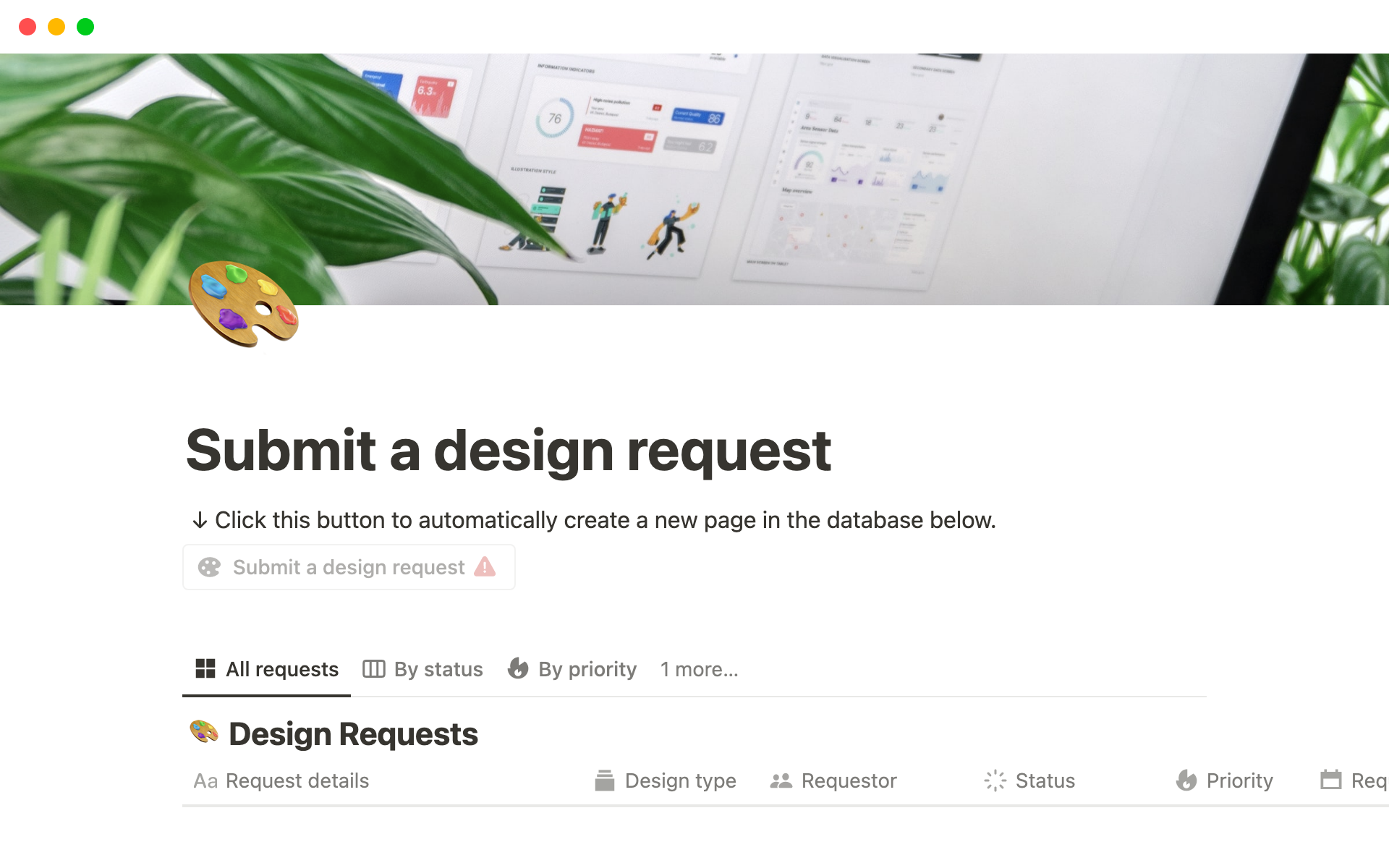A screenshot, seemingly taken from a Mac, showcases a user interface. The top of the image has a white banner featuring the characteristic red, yellow, and green traffic light icons on the left side. The central part of the screenshot presents a workspace with artificial green plants positioned on both the left and right edges, simulating a desktop aesthetic.

In the middle of the workspace, there is a paint palette, colored in brown, holding small splashes of purple, light blue, green, yellow, and red paint. Below this, there's prominent black text on a white background that reads, "Submit a Design Request." Beneath the heading is a down arrow and a directive text explaining, "Click this button to automatically create a new page in the database below."

Further down, a white rectangle with a gray border features another paint palette icon and invites users to "Submit a Request." Adjacent to this box is an unexplained caution sign.

Below it, the text "All Requests" appears in black, followed by gray text options: "By Status," "By Priority," and an ellipsis indicating more options. This section is completed with another colorful paint palette icon.

Finally, the section titled "Design Requests" is displayed in black text, followed by gray text detailing "Request Details." The categories listed include "Design Type," "Requester," "Status," "Priority," and "Reg." The entire interface is neatly presented, with no additional elements beyond this point.